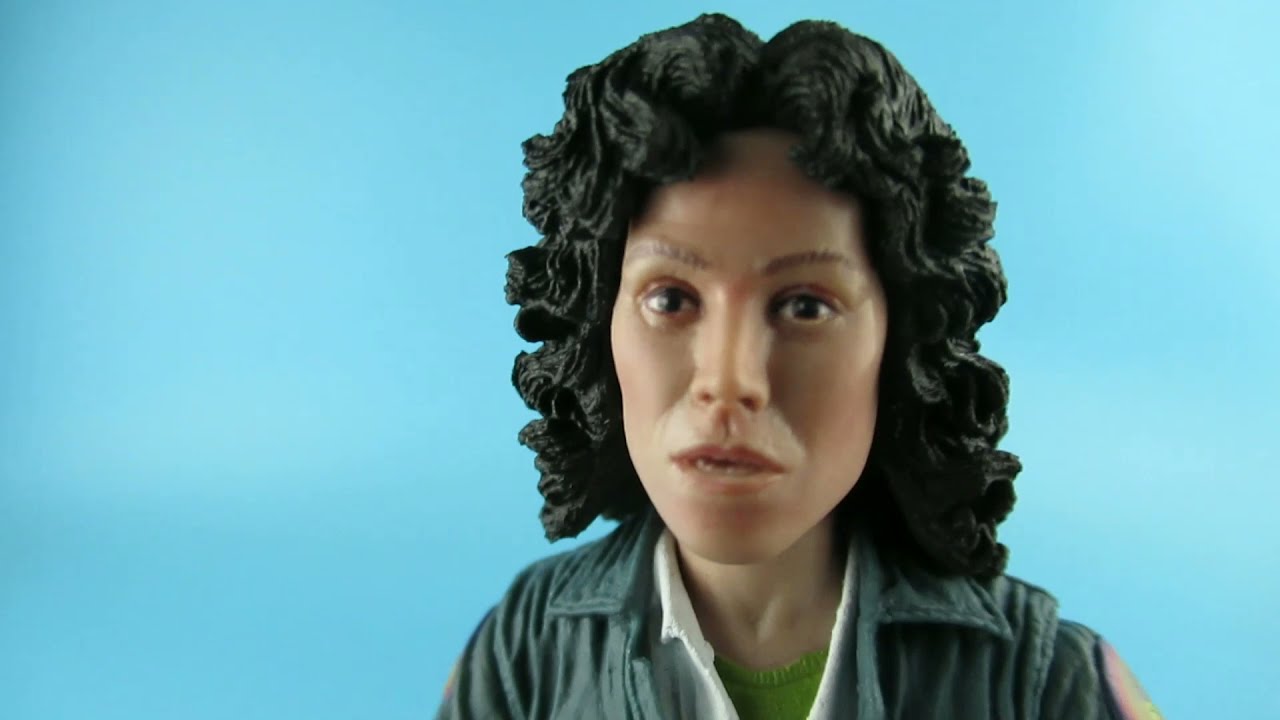The image features a highly realistic, claymation-style figure of a middle-aged woman with curly black hair, posed against a gradient aqua-blue background that transitions from lighter in the center to darker at the edges. This lifelike animated figure, possibly resembling the protagonist from the "Alien" franchise, has a quizzical expression with wide-open dark brown eyes and a slightly open mouth. The figure, appearing to be a light-skinned or light color Hispanic woman, is dressed in a layered outfit: a green collared shirt or jacket with a patch on the left shoulder, a white open-collar shirt underneath, and a green tunic or t-shirt. The attention to detail includes light brown eyebrows and subtly painted plastic features, such as the hair and skin-colored paint on the collar, enhancing the figure's realistic yet unmistakably artificial appearance.